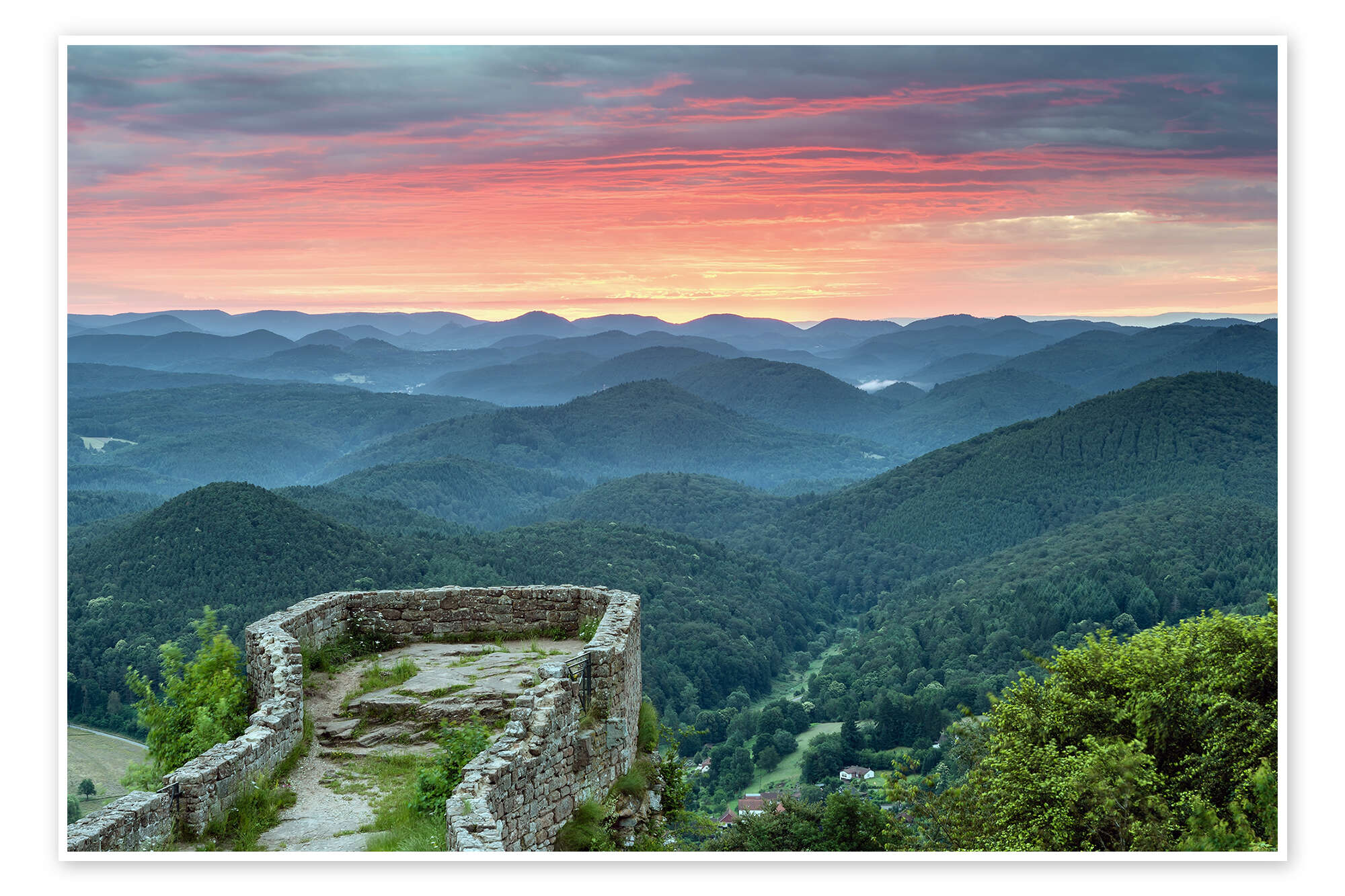The image, a horizontal-rectangular painting or photograph, showcases a mesmerizing mountain scene viewed from a high vantage point. In the foreground, there is a stone viewing area akin to a brick wall, possibly reminiscent of an old building or the Great Wall of China, where visitors can stand and admire the landscape. Stretching out below are the tops of dark, abstract mountains shrouded in green vegetation and some fog, creating an almost surreal impression. The expansive valley, dotted with dense forests of dark brown trees and a few scattered cottages, extends into the distance, gradually fading to a purplish hue due to atmospheric perspective. The scene is bathed in the warm, transitioning colors of sunset, with the horizon glowing in red and orange, and the sky above transitioning to a darker shade, gently interspersed with calm clouds.